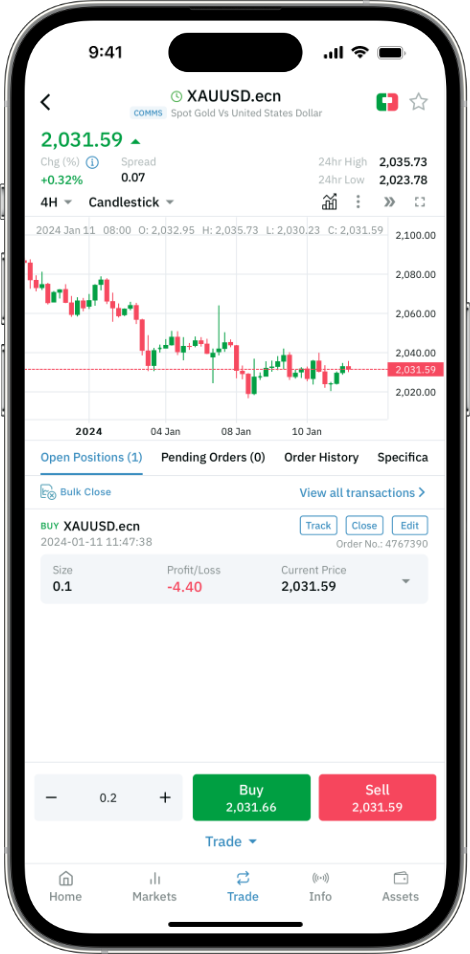The image depicts a smartphone screen displaying a real-time stock performance chart for the stock symbol "XAUUSD.ECN," which represents the spot gold price against the United States dollar. At the top of the screen, the stock symbol and its corresponding description are visible: "spot gold versus United States dollar." Directly below this, the current price is listed as $2,031.56, highlighted in green with an upward triangle indicating a positive change. Below the current price, a section labeled "CHG% Spread" provides further details: "CHG" shows a percentage change of +0.32%, also in green, while "Spread" is recorded as 0.07.

To the right of these values, the stock’s 24-hour high and low prices are displayed, with the 24-hour high at $2,035.73 and the 24-hour low at $2,023.78. Beneath this summary, the image features a candlestick chart with fluctuating green and red bars representing market trends and price changes over time.